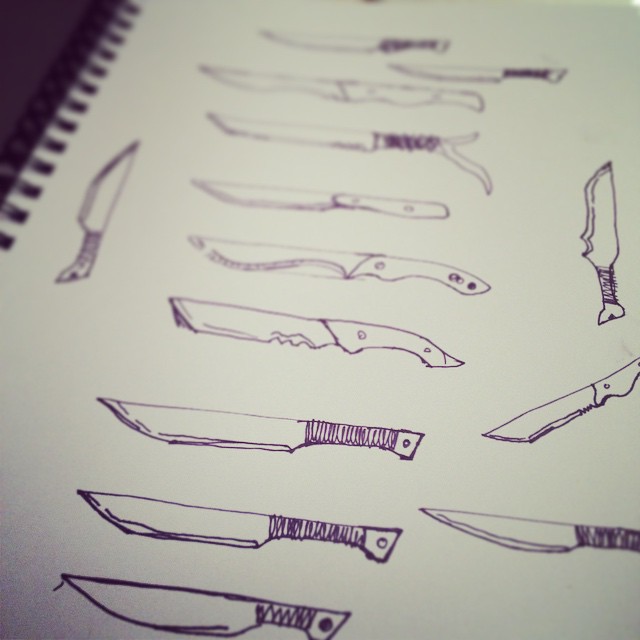This photograph captures a spiral-bound sketchbook with its coiled binding visible in the upper left corner. The sketchbook is opened to a page filled with an array of pen and ink drawings of various knives, rendered in purple ink. The knives, a total of about 16, predominantly resemble hunting or pocket knives and feature distinct single-bladed designs. They are arranged mostly horizontally, pointing to the left, while a few on the right and one on the left side point upward or at different angles. The focus of the photograph is sharper on the lower third, emphasizing the bottom three knives, whereas the sketches at the top appear blurred. The handles of these knives are minimally detailed; however, there are instances of shading and intricate designs, such as one handle forked into a shape resembling the letter 'B' and others featuring corded grips. The image overall has a subtle black and purple hue, adding a unique tint to the white sketchbook page.